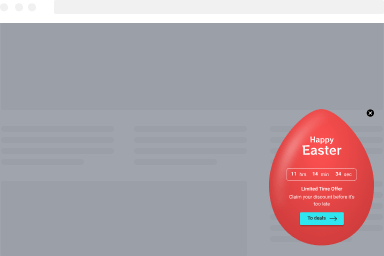A grayed-out web page features a minimalist design with various elements dispersed across the screen. The entire page is bathed in gray tones, providing a subdued backdrop. In the bottom right corner, a striking red egg marked with the words "Happy Easter" in white letters stands out vividly. 

Adjacent to the egg is a small white text that is barely legible due to its tiny size. Dominating the lower section is a horizontal rectangle displaying the countdown "11 HRS, 14 MIN, 34 SEC" in bold figures, indicating elapsed time. Beneath this timer, the green text reads "UNLIMITED TIME OFFER" followed by another line that says "Own your [illegible text] before it's too late."

A large blue button below this message catches the eye with an inscription in black font that is partially unreadable, accompanied by a right-pointing arrow. 

Across the center of the gray rectangle, there are several lighter gray rectangles aligned in a row, each segmented by thin, darker gray lines creating a grid-like effect. At the very top of the webpage, a simple navigation bar is located, featuring three dots in the upper left corner suggestive of a menu or additional options.